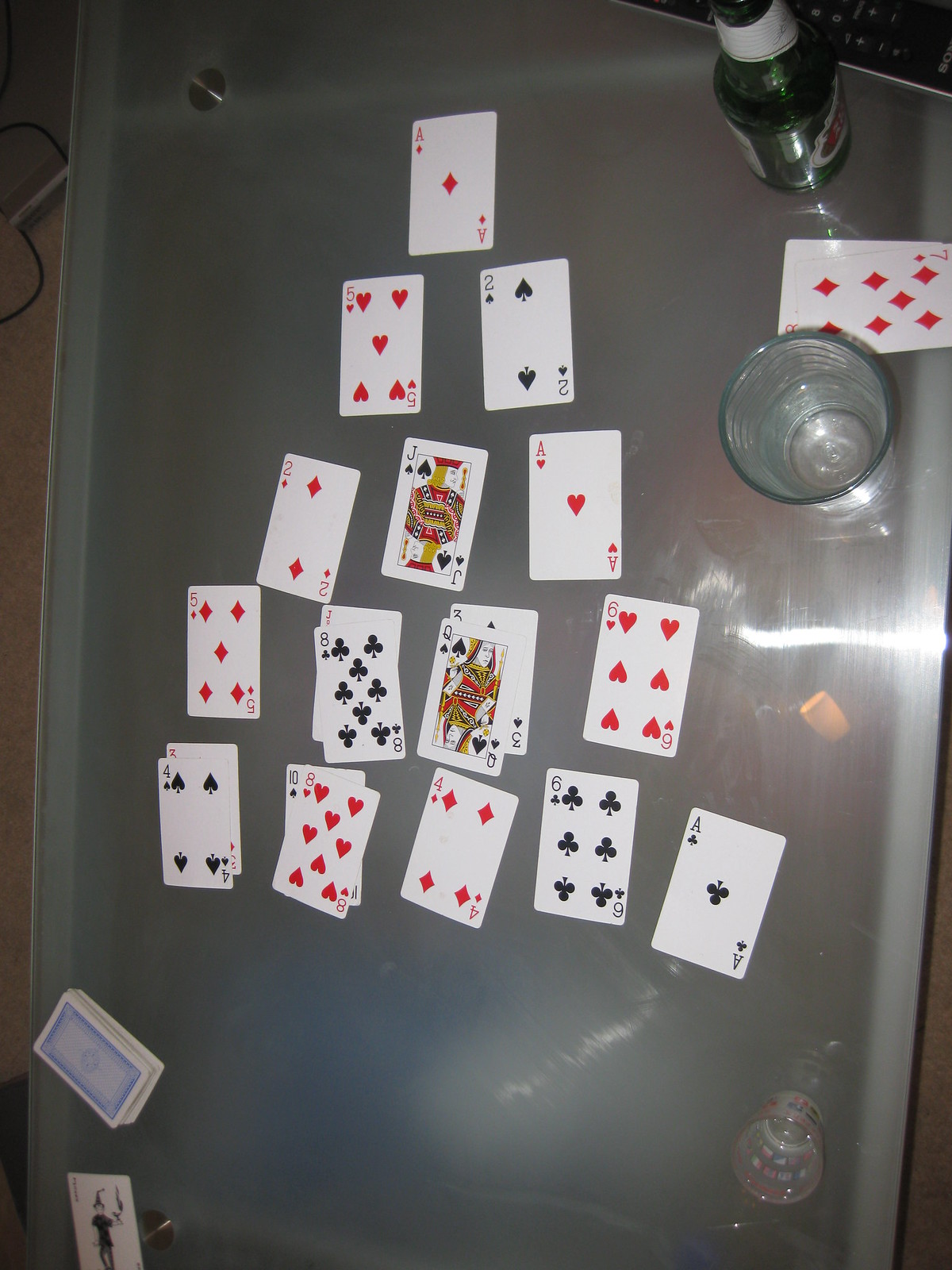This overhead photograph captures a sleek, metallic tabletop reflecting the ambient light. Central to the image is a meticulously arranged pyramid of playing cards, indicative of a game of solitaire in progress. The pyramid features five descending rows, each row expanding by an additional card. At the pinnacle of the pyramid is the Ace of Diamonds, complemented by the Ace of Hearts and the Ace of Clubs interwoven below. 

Adjacent to the pyramid, on the right side of the table, a hand of cards rests with the Seven of Diamonds prominently on top. Below the setup lies a neatly stacked deck of cards, seemingly ready for the next draw. 

Accompanying the game, two glasses and a bottle add a touch of casual leisure to the scene. One is a shot glass and the other, a larger beer glass, both positioned next to a beer bottle, suggesting a laid-back atmosphere.

The interplay of the reflective tabletop and the detailed card arrangement, along with the presence of the beverages, creates a vivid snapshot of a solitary game in a moment of quiet relaxation.